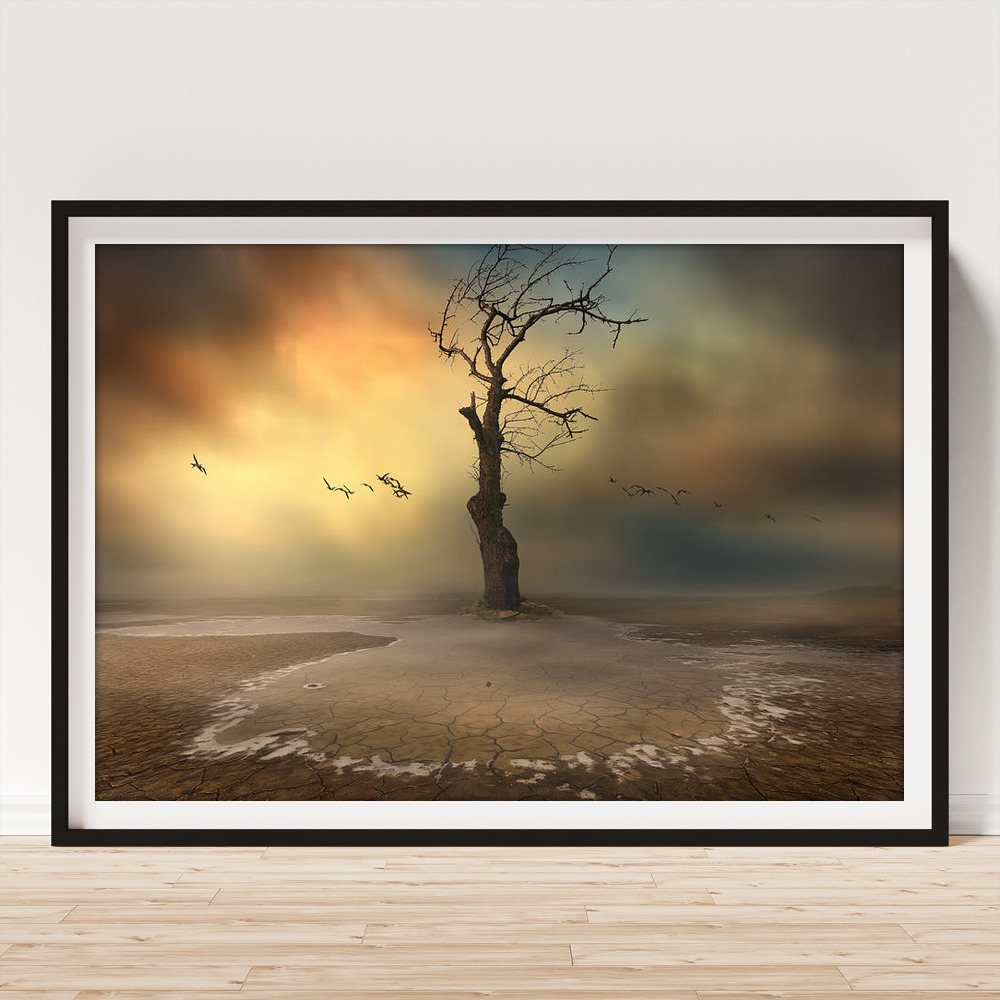This is a photograph of a framed poster leaning against a white wall on a light, hardwood floor. The poster is encased in a black frame with a white matting. At the center of the photograph is a barren tree with thin, twig-like branches, devoid of leaves, standing on parched, cracked, and brown earth. Surrounding the base of the tree is a white salt-like film. The background features a blurred sky in a mix of yellow, black, and gray shades, with a hint of blue and orange suggesting a covered sun. A line of indistinct black birds flies across the sky. The overall color palette consists of yellows, browns, tans, blacks, and some reddish hues, giving the image a beautiful yet dreary atmosphere. There are no people or text in the photograph. The poster appears to be marketed for sale online.